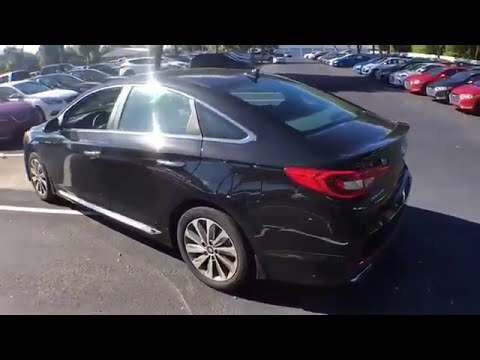This horizontally aligned, small-sized rectangular photograph features prominent black borders at the top and bottom, framing a detailed side view of a four-door black car parked in a lot. The car, likely a BMW, is shown from the left side, capturing part of the rear and the driver's side with its window down, revealing the steering wheel. The sunlight casts strong reflections off the back window and the car's glossy black surface, contributing to a very shiny and glary appearance.

The vehicle is positioned diagonally, parked improperly over the white lines marking the parking spaces on the medium gray pavement. Surrounding the car, the scene reveals a bustling parking lot filled with various cars, including red, black, white, and even some maroon vehicles. Rows of cars extend to the horizon on both the upper left and upper right sides of the image. The background includes hints of a white rectangular building in the upper right corner and some scattered trees far off in the distance, framing the busy, brightly lit environment of either a shopping center or a car dealership lot.